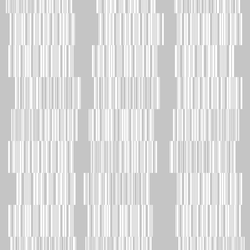The image depicts a light gray square featuring a series of short, vertical, dark gray and white lines, reminiscent of barcodes. These lines are veined and slightly offset from each other, creating a staggered pattern where each row is misaligned just a little to the left or right of the one below it. The lines are arranged in three columns and nine rows, with the overall appearance having a robotic or barcode-like quality. The meticulous alignment and repetitive nature of the lines provide a structured yet slightly disordered aesthetic within the monochromatic scheme.